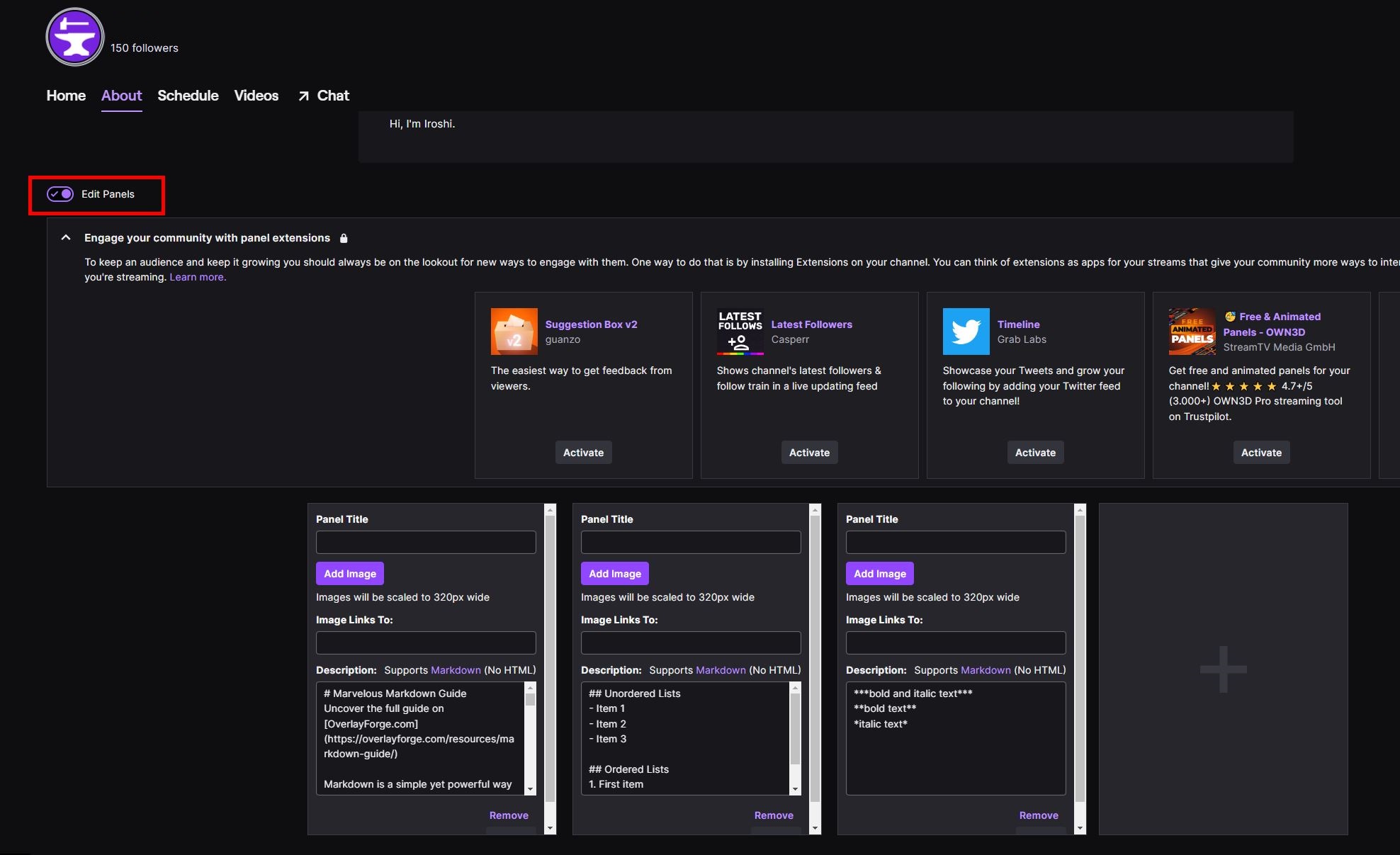This image depicts a computer screen featuring a page with a dark black background, which is a consistent theme throughout the smaller windows and elements within the image. Starting at the top left corner, there is a circular emblem resembling a blacksmith's insignia, with a white hammer and anvil icon set against a purple background. Beside this emblem, it shows '150 followers' in white text.

To the right of these elements is a horizontal navigation list in white text, which includes the options: "Home," "About," "Schedule," and "Videos." An arrow pointing diagonally upwards to the northeast directs attention to the word "Chat." The "About" tab is underlined and highlighted in a lighter purple, indicating that this is the active page.

In the central area, a prominent black rectangular box contains the greeting "Hi, I'm Iroshi," written in white letters. Beneath this greeting is a highlighted box with a red border and a checkmark inside a purple circle, labeled "Edit Panels" in white text. Below that, there's a message encouraging user interaction: "Engage your community with panel extensions," followed by a detailed description.

Further down, the page displays four horizontal boxes, each with a black background and distinct emblems. The first box, titled "Suggestions Box V2," features a V2 emblem on an orange background. The remaining three boxes, labeled "Panel Title," provide space to add images and image links, along with additional informational descriptions. At the bottom, there is a blank box with a plus sign, suggesting that more panels can be added.